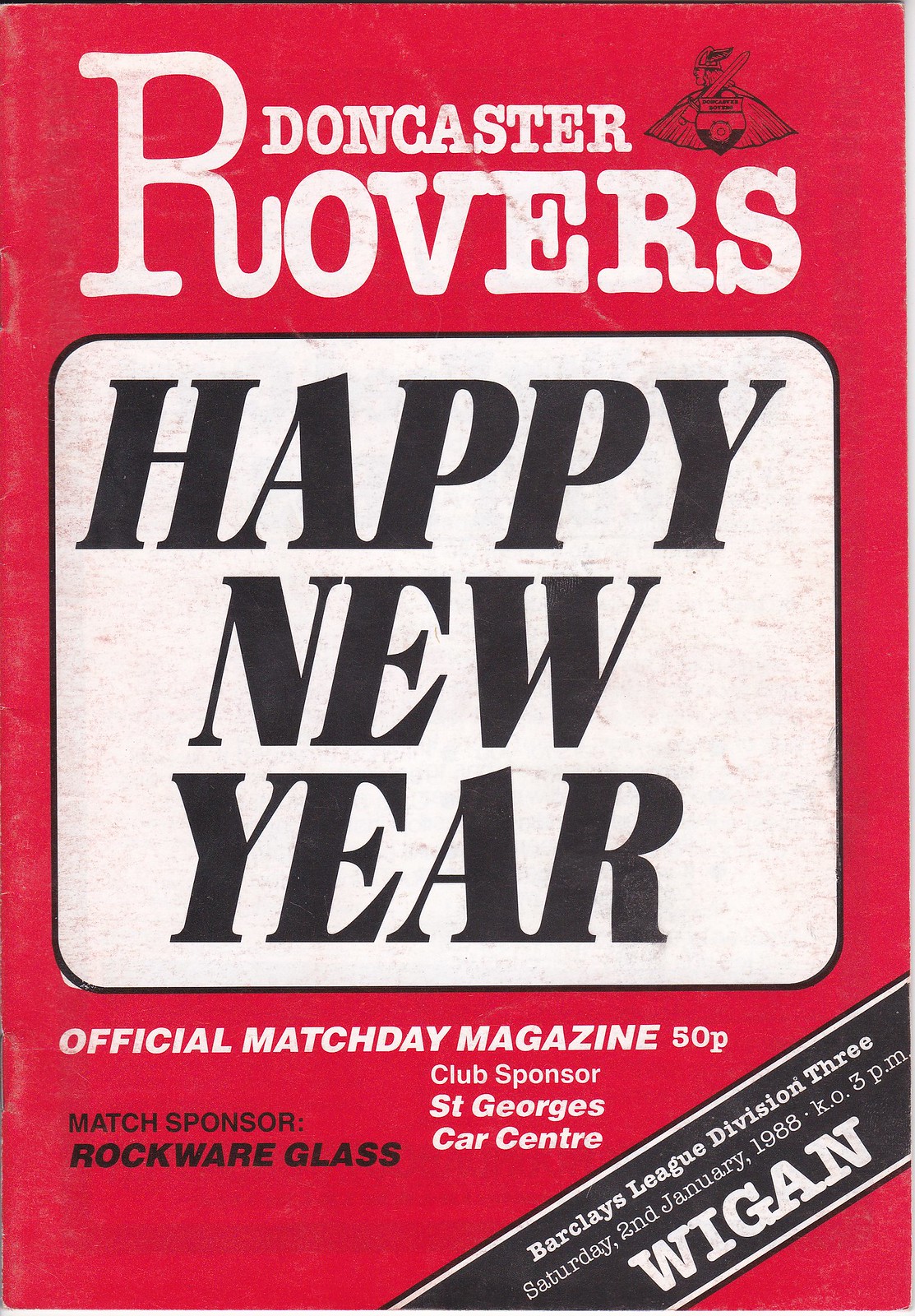This vintage 1988 Doncaster Rovers Match Day magazine cover features a predominantly black-and-white design accented with a striking red background at the top. The bold, white text at the top reads "Doncaster Rovers," with a large, extended "R" in "ROVERS" and a team logo of a warrior with a shield and sword to the right. Centered on the cover is a soft-edged white rectangle with the phrase "Happy New Year" in large, italic black text. Below this, white italic bold text announces that it is the "Official Match Day Magazine" priced at 50p. The bottom half of the cover includes details of the club sponsor, St. George's Car Center, and the match sponsor, Rockwear Glass. In the bottom right corner, a black banner with white text provides match details: "Barclays League Division III, Saturday 2nd January 1988, K.O. 3 p.m., Wigan." The publication style is distinctly vintage, capturing the essence of its time.